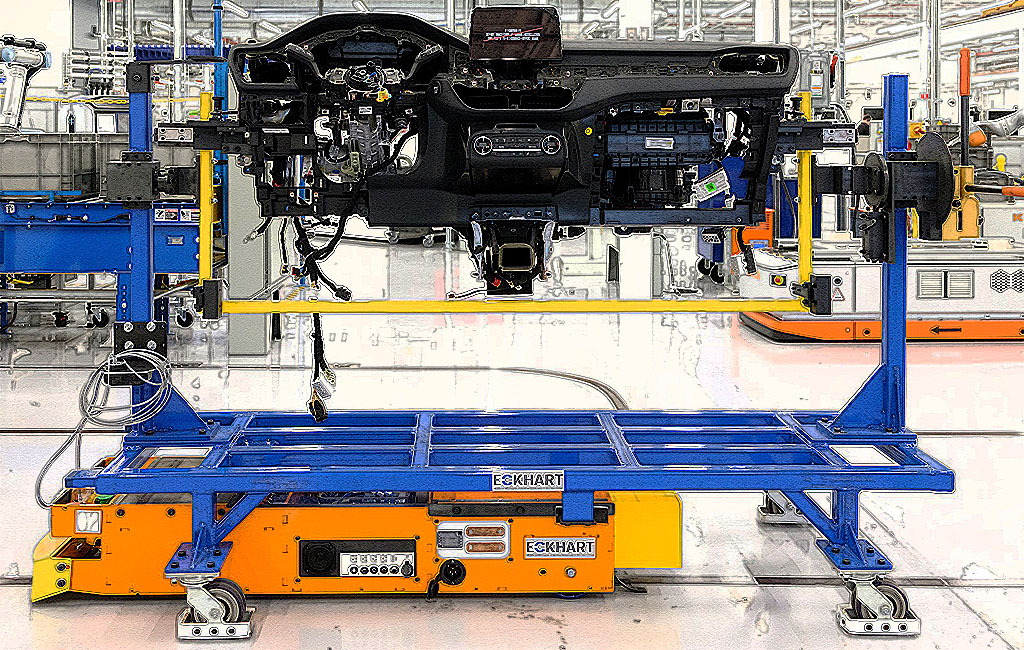This detailed image captures a bustling factory floor, primarily focused on a sophisticated assembly setup. Dominating the foreground is a blue metal lift on wheels, securely locked in place, positioned beneath an intricate piece of machinery. This machinery features an orange control panel at its base, clearly identified as an Eckhart system. 

The lift hoists an exposed vehicle dashboard, revealing the inner components of a steering wheel on the left, a central area possibly housing a stereo, and an upper section likely designed for dash-mounted screens. The facing of this dashboard has been stripped away, granting a clear view of its internal structure and components, including several holes that might be for light fittings.

In the background, the scene expands into a large factory space lit by expansive warehouse lighting. Numerous other mechanical tools and tables are scattered throughout, complemented by shelving units and various equipment in hues of silver, blue, yellow, white, and black. The environment appears almost stylized, with a somewhat blown-out effect enhancing its industrial ambiance.